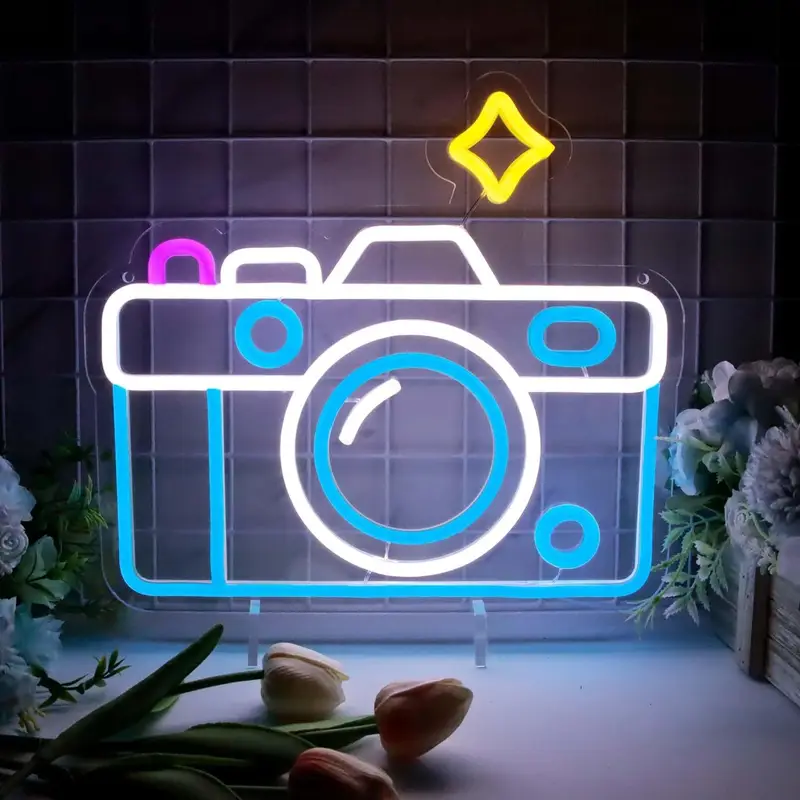This image, which appears to be either a realistic photograph or a computer-manipulated picture, features a neon sign designed as an outline of a camera. The camera sign is illuminated in white, blue, and purple neon, with a small yellow star above it, possibly representing a flash. This neon sign is mounted against a black wall with a grid pattern, and the scene is lit predominantly by the neon light. The ground surface in the image is stark white, enhancing the contrast. In the foreground, there are three light pink tulips with green stems lying on the white surface. Additional assorted flowers are present on both the left and right sides of the image, possibly hinting at a florist's touch. The overall ambiance suggests that this could be a showcase in a florist shop, with the flowers accompanying the neon camera as a prop, or a creative setup for a photography studio.